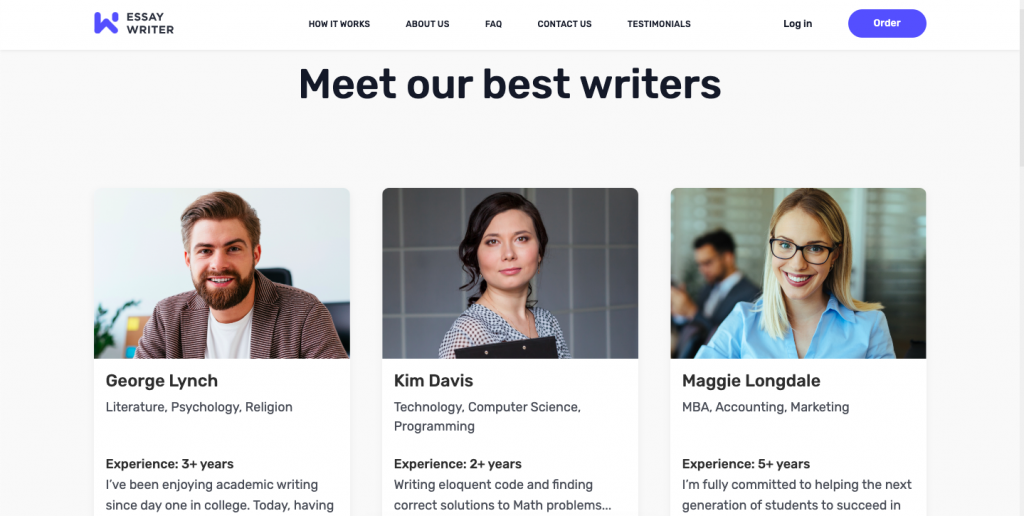The image features a white top border with a blue logo resembling the letter 'W' and the text "Essay Writer" next to it. Adjacent to this, there are navigation links labeled "How It Works," "About Us," "FAQ," "Contact Us," "Testimonials," and "Login," followed by a blue "Order" button. Below this header, a gray box displays prominently in large bold black letters: "Meet Our Best Writers."

On the left side of the gray box, there is a photograph of a man seated in a chair, facing the camera. The background includes a plant and some scattered papers. The man, identified as Jordan Lynch, has a beard, goatee, and mustache, and is wearing a white shirt paired with a brown suit jacket. His caption reads: "Jordan Lynch, Literature, Psychology, Religion. Experience: 3+ years. 'I’ve been enjoying academic writing since day one in college.'"

To the right of Lynch’s profile is another section featuring Kim Davis. The text lists her areas of expertise as "Technology, Computer Science, Programming" and mentions that she has "Experience: 2+ years." Her caption states: "Writing elegant code and finding correct solutions to math problems."